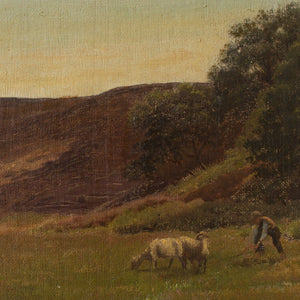This image appears to be an old, grainy wilderness painting capturing a pastoral scene. At the center, a small figure, possibly a child or young man, is bending down and appears to be coaxing or herding a couple of tiny sheep with some white and brown fur towards him. He is dressed in brown attire, possibly western in style, and might be wearing a hat. The sky above is a mix of light blue, gray, and orange hues, decorated with clouds, indicating an early fall or late spring setting. To the far right stands a large tree with many green leaves, and near it, a smaller tree with brown branches. The background features a rocky hill and a valley of brown dirt that transitions into a meadow covered in green pasture. The rich green foliage and the earthy hues of the landscape create a serene, rustic atmosphere, anchoring the human and animal elements within the timeless beauty of nature.